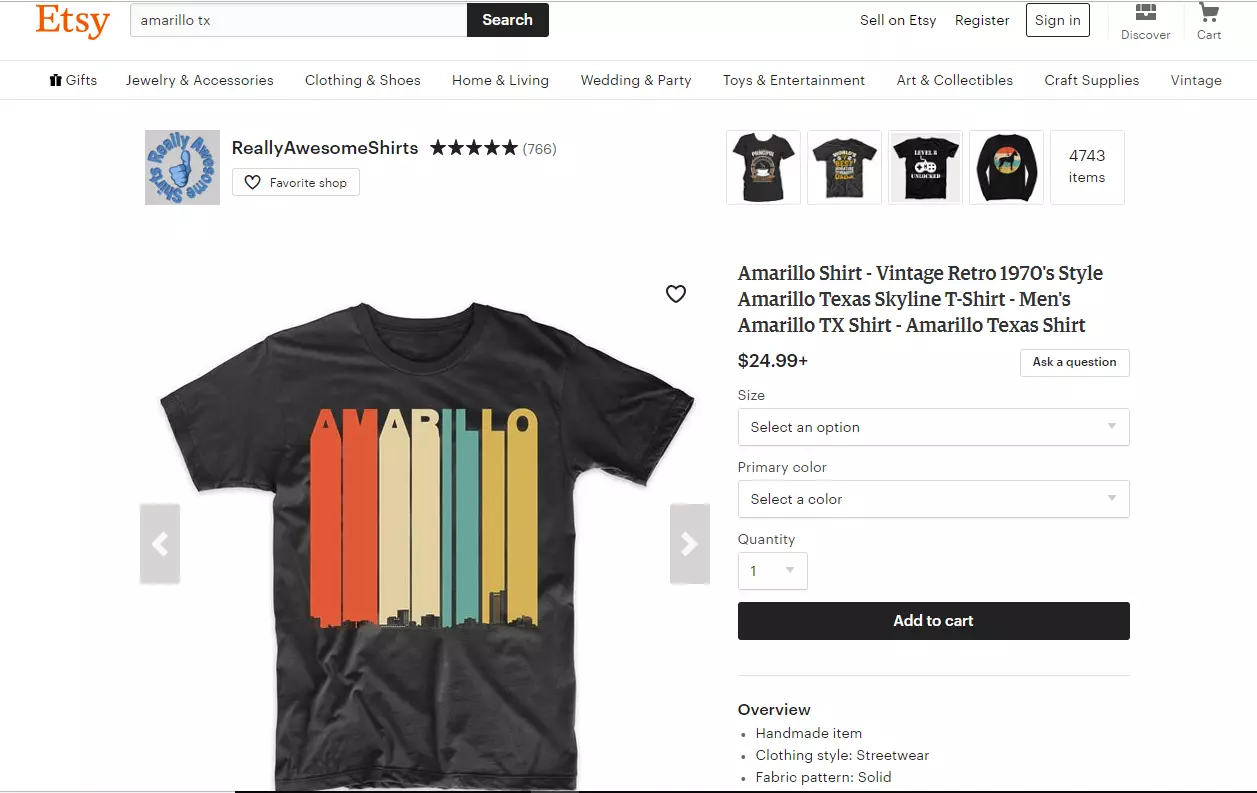In the image, there is a detailed view of an Etsy shop specializing in vintage and handmade items. The shop seems to be highly rated with a prominent five-star rating and labeled as a "favorite shop." Spread across the white background, there are various categories listed such as gifts, jewelry, accessories, clothing, shoes, home and living, wedding and party, twins, intimate items, art and collectibles, classifieds, and vintage.

The focus is on a series of vintage-style shirts, predominantly black with unique designs and graphics. The shirts displayed include four distinct black shirts, each described in detail:

1. Amarotex black shirt featuring a vintage red jar resembling a 1970s style.
2. Amarotex discounted men's t-shirt priced at $24.99.
3. Handmade shirt options with rubber color customization.

Among these, there is a striking red shirt with the word "Amarillo" in large letters. The letters seem to be melting or dripping down, creating a visually captivating effect. The items have a price tag of $35.00 each and are available in different styles and colors, including gray.

Overall, the image showcases an eclectic mix of fashion items with a vintage flair, emphasizing high-quality handmade craftsmanship and unique design elements.